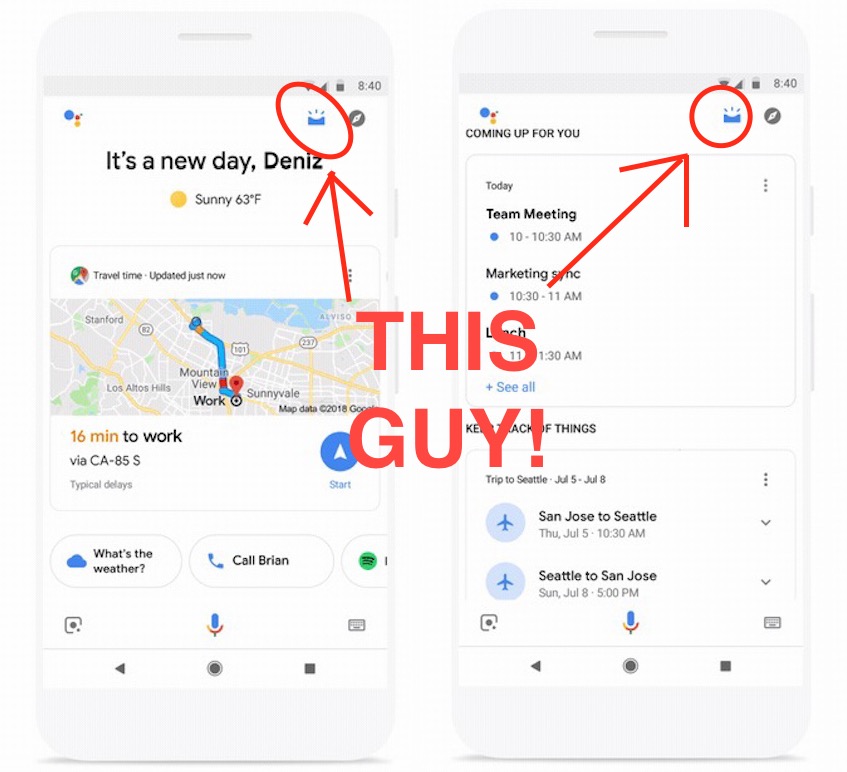The image depicts two cell phones displaying simulated search results. The focal point is a digitally added phrase in red text at the top of the image that reads "THIS GUY!" accompanied by an exclamation point. Both cell phones feature a unique blue icon resembling a rectangle with an indented top and three small lines extending from it; these icons are circled and highlighted with red digital arrows pointing to them.

On the first cell phone, the display reads "A New Day DENIZ," indicating the weather conditions as sunny with a temperature of 63 degrees Fahrenheit. The screen also shows a map with directions, stating "16 minutes to work via CA-85S" and noting "typical delays." Additionally, there is a "Start" button for navigation. The bottom of the screen has several buttons, including options like "What's the weather," "Call Brian," among others.